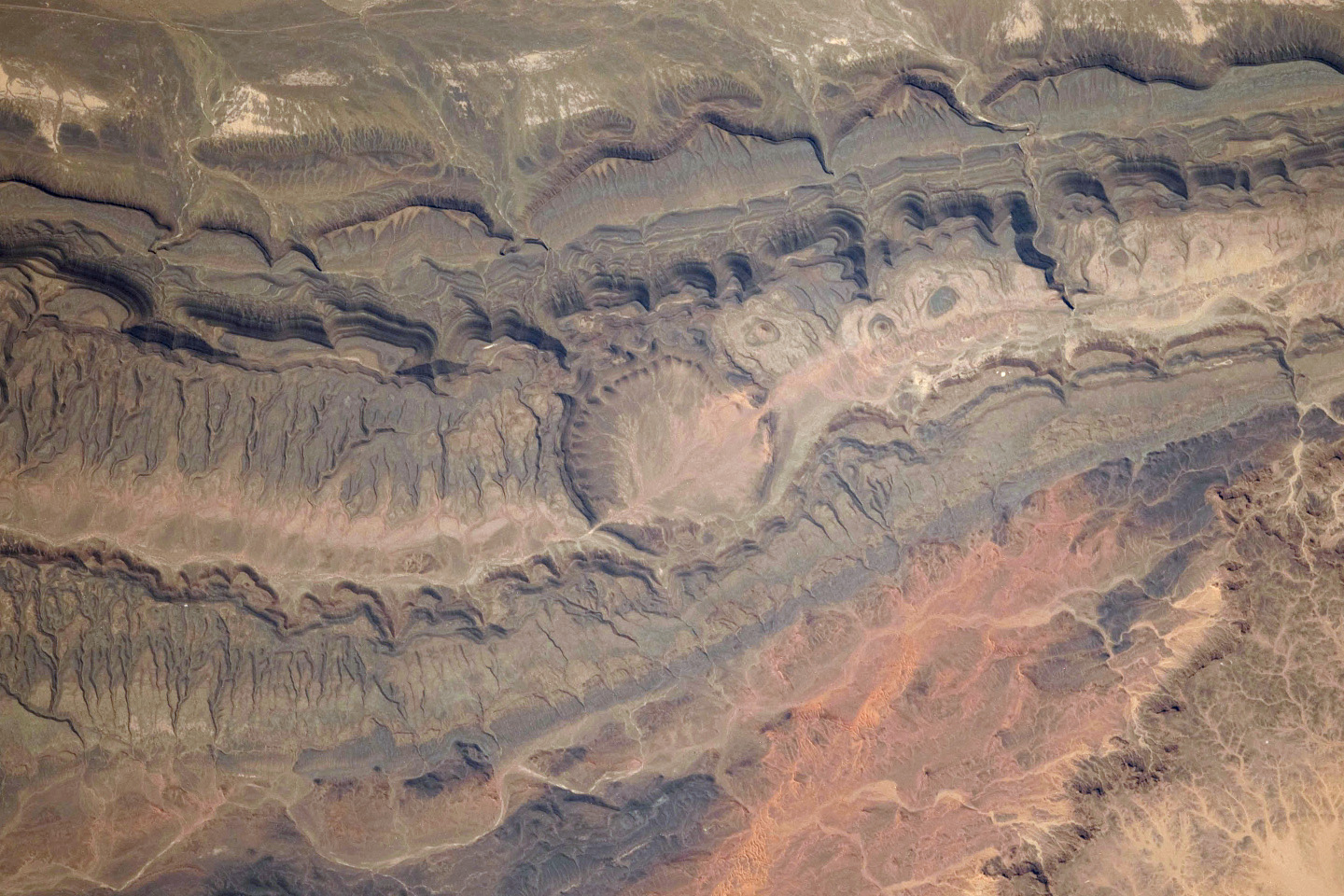This high-altitude or possibly satellite image showcases a fascinating and intricate landscape, characterized by its wavy, veined appearance. The terrain below, which could be either a deserted landmass or an alien-like surface, features a mix of green and dark gray hues. The top section of the image reveals medium brown, almost raised formations with patches of white, suggesting either soil variations or eroded areas. Moving towards the bottom, the landscape dips, displaying darker brown tones, perhaps indicative of dried-up lakebed remnants or rock formations. A circular shape lies near the center, adding to the mysterious, vein-like patterns that stretch across the image, reminiscent of water flow pathways or geological veins. This visually compelling and desolate scene, devoid of any human elements, leaves an impression of it being from Earth or possibly even another planet.